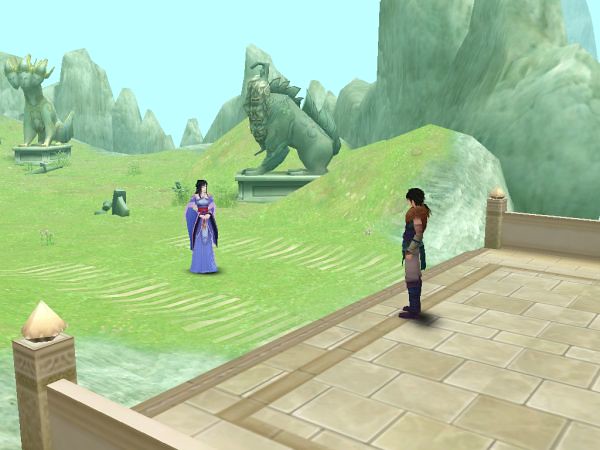This image captures a dynamic moment from live gameplay, possibly taken from a device such as a gaming PC, phone, or TV. The scene showcases two characters positioned on opposing sides of a bridge. On the right, a male character clad in brown clothing stands firmly on the brown and white structure of the bridge. Across from him, on the left side of the image, a female character with flowing black hair is dressed in a striking purple dress, standing on a lush green field. The backdrop features an expansive landscape adorned with dramatic, pointy mountains extending to the left, setting a majestic and immersive scene. Adding to the mythical ambiance, three-headed animal figures can be discerned in the background, contributing to the game's fantastical atmosphere.